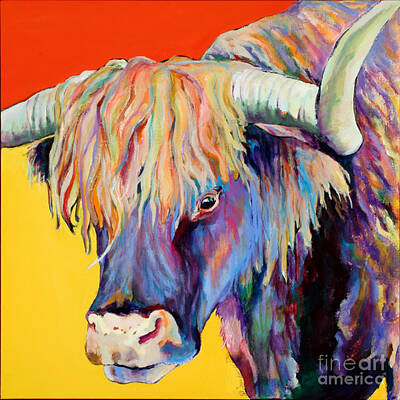This vibrant painting, which prominently features a bull, is richly adorned with a spectrum of colors. The bull's head is the primary focus, depicted in a three-quarter view facing to the left. The horns, long and sharp, are primarily white with hints of purple and orange, resembling those of a Texas longhorn. The bull's dense hair cascades over its forehead, nearly obscuring its dark, black eyes. The fur is a kaleidoscope of colors, including blue, yellow, green, purple, red, dark pink, and turquoise. The snout is a lighter cream color. The background consists of a solid red upper section and a solid yellow lower section, adding to the image's boldness. In the lower right corner, the watermark "Fine Art America" is visible, indicating the artwork's origin. Overall, the piece evokes the playful and dynamic spirit of fine art through its vivid and varied hues.